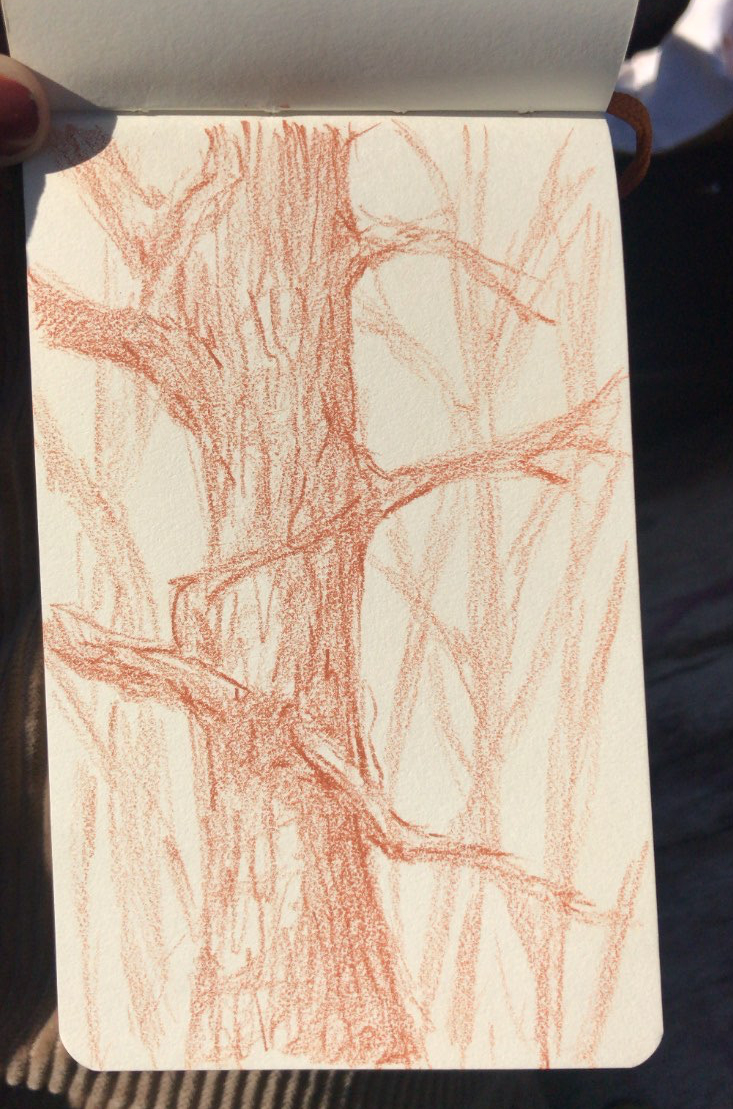The image features a colored pencil drawing of a tree, predominantly rendered in a rusty orange or brownish-red hue, on a vertically-opened notepad or drawing pad. The drawing, held up by a hand with reddish nail polish on the thumb visible in the upper left-hand corner, presents a tree trunk with numerous thin branches extending from it. Notably, the tree lacks leaves, emphasizing the bare quality of the branches. The background of the image itself showcases a clutter of smaller tree trunks or bush-like lines, adding depth and a sense of natural complexity to the scene. The drawing sheet shows a hint of the previous page at the top, indicative of its position in the notepad.